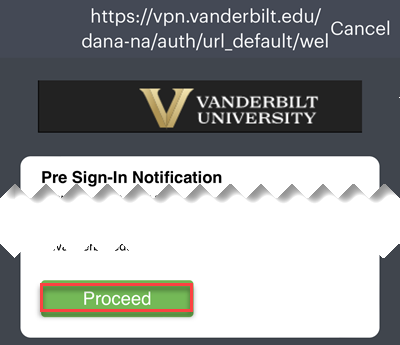This image appears to be a screenshot from a digital device, possibly a computer or a smartphone, displaying a login or notification page. The background is a dark gray color. At the very top of the image, in white script, the URL "https://vpn.vanderbilt.edu" is repeated three times.

In the upper right-hand corner, there's a "Cancel" button. Directly below the repeated URL, there is a prominent black rectangle featuring a large gold "V" next to which are the words "Vanderbilt University" in white text.

Below this black rectangle, there is a white rectangle with scalloped edges along the top and bottom, labeled "Pre-sign-in notification." The scalloped design looks as though someone cut out portions of the information, leaving a few words visible on the left side through three of the scalloped points.

Near the bottom left corner of the white rectangle, there is a green button with the word "Proceed" written in white text. This button is highlighted by a red rectangle that has been added to draw attention to it. There are no back buttons or additional navigation options visible in the image.